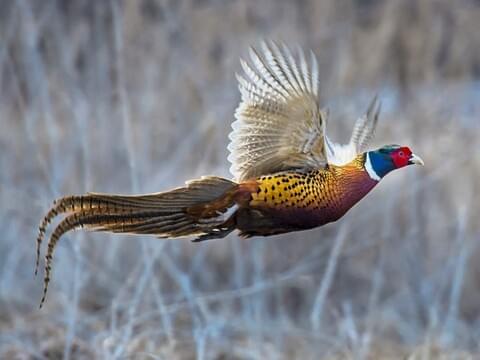This is a color photograph taken outdoors showcasing a ring-necked pheasant in mid-flight, occupying about 85% of the image. The background is a blur of tall, dry brown grass, emphasizing the bird as the central focal point. The pheasant's wings are extended and appear predominantly white, with possible black outlines. Its long, flowing tail feathers are brown, hanging down elegantly as it soars. The bird's body is a tapestry of vibrant colors: the upper chest is a deep brown transitioning to shades of yellow on the stomach, adorned with black speckles. The pheasant’s head and neck are notably colorful, with a distinct white band encircling the neck, followed by iridescent blue feathers that blend into green at the top. The face is a striking red, contrasting sharply with the white beak, which has a black tip. The legs of the pheasant are tucked neatly underneath its body, completing the graceful airborne pose. Overall, the bird's vivid plumage and dynamic posture create a stunning and detailed image of this strikingly beautiful creature in motion.